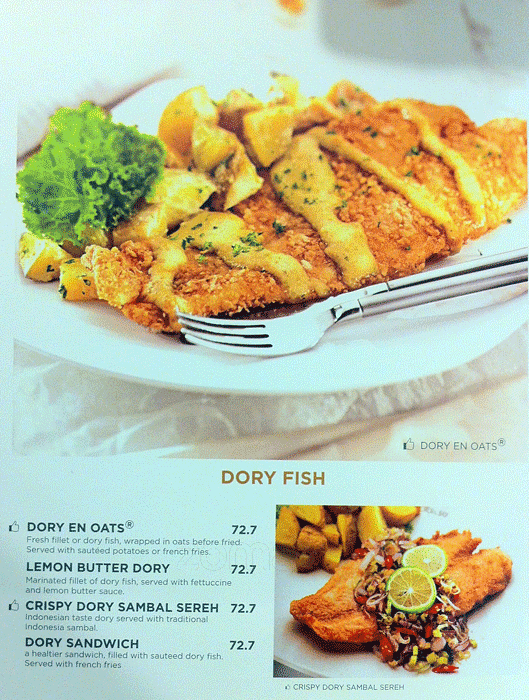The image displays a page from a menu, primarily featuring a large photo of a dinner entrée on a white plate. The dish appears to be a piece of fried dory fish with a crumb coating, drizzled with a yellow sauce, and accompanied by sliced or roasted potatoes and a sprig of parsley or kale as decoration. Resting on the bottom part of the plate is a stainless steel fork. Below the main photo, there is a text box with menu details. The highlighted menu items, each priced at $72.7, are: 'Dory and Oats,' a fillet of dory fish wrapped in oats and fried, served with sautéed potatoes or french fries; 'Lemon Butter Dory,' a marinated dory fillet with fettuccine and lemon butter sauce; 'Crispy Dory Sambal Sereh,' infused with Indonesian sambal and served with traditional Indonesian sambal; and a 'Dory Sandwich,' featuring sautéed fillet in a healthier sandwich option with french fries. There is also a thumbs-up symbol next to 'Dory and Oats' and 'Crispy Dory Sambal Sereh.' An additional smaller photo shows a fried dory fillet topped with a corn and tomato chutney, garnished with lime and lemon slices, labeled as 'Crispy Dory Sambal Sereh.'